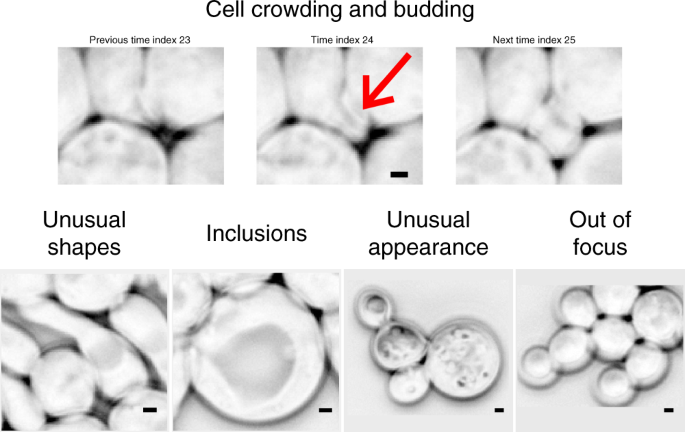This detailed image, presumably from a textbook or educational slideshow, showcases a collage of black and white photographs of cells under high magnification, distributed in two rows. The background is entirely white, providing a stark contrast to the dark cell images. The top row features three images labeled under the heading "Cell Crowding and Budding." These images are a sequence showing the progression of cellular activity: the first image is tagged "Previous Time Index 23," the second (center) image, highlighted by a red arrow pointing to a specific part of a cell, is marked "Time Index 24," and the third image is labeled "Next Time Index 25." Below these, the bottom row presents four distinct images, each with their respective labels in black text. From left to right, they are titled "Unusual Shapes," displaying multiple clustered cells; "Inclusions," featuring a large cell surrounded by smaller ones; "Unusual Appearance," with three small cells and one larger cell; and "Out of Focus," where the cluster of cells lacks clear visibility. Each cell image appears slightly blurred, consistent with microscopic examinations, and the structures predominantly exhibit circular forms.